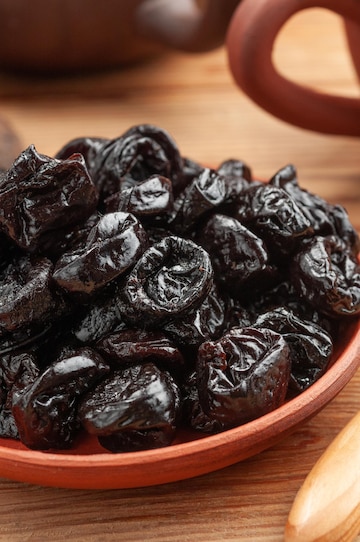In the image, a shallow red dish, deeper than a plate but shallower than a full bowl, is prominently displayed in the foreground, filled and slightly overflowing with dried fruits that resemble prunes. These prunes, likely dried cherries or plums, are a deep purplish-black color and exhibit a wrinkled, indented appearance, typical of desiccated fruits. The prunes are stacked about two inches high and some show concave surfaces suggesting they are shriveled and dried. This dish, which sits atop a medium wood surface that could be a table, adds a rustic charm to the setting. In the background, the top right corner showcases a red cup handle next to what appears to be another handle from a separate cup. Additionally, the bottom right corner hints at a protruding piece of wood, possibly part of a wooden spoon. The overall well-lit and clear composition of the picture highlights the attractive arrangement and texture of the prunes, making the scene appealing and detailed.